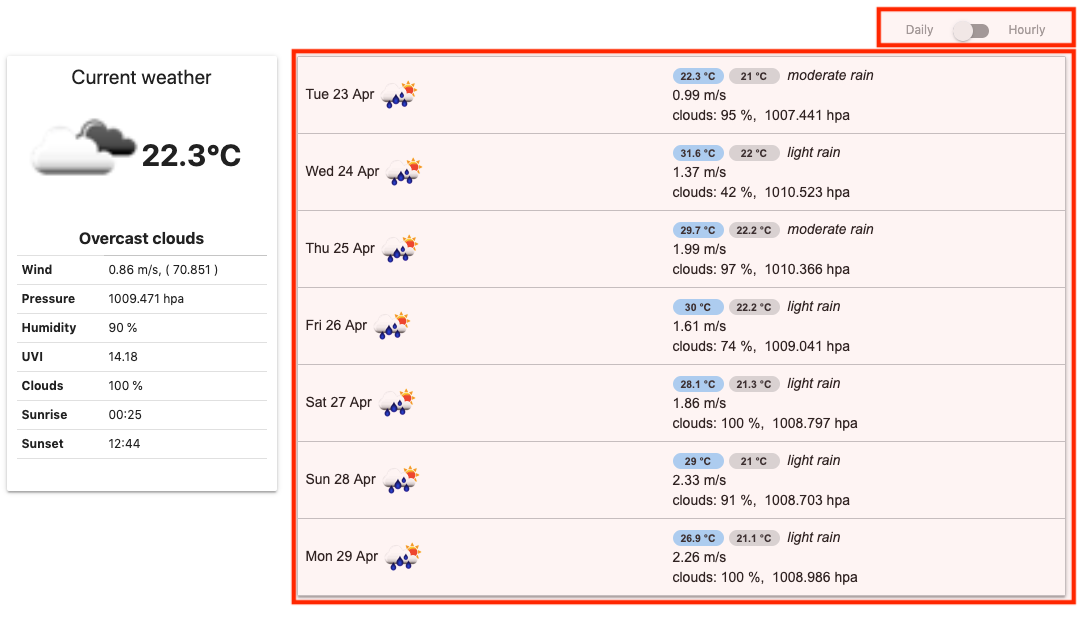A detailed photograph of a weather application interface is presented. On the left side, the current weather conditions are displayed in a white box bordered by a red square. The current weather section includes graphical representations of a white cloud and a gray cloud, indicating overcast skies. The temperature reads 22.3 degrees Celsius. Additional meteorological details provided include: wind speed at 0.86 meters per second, atmospheric pressure at 1,009.471 hPa, humidity at 90%, ultraviolet index (UVI) at 14.18, and cloud coverage at 100%. The times for sunrise and sunset are listed as 00:25 and 12:44, respectively.

At the top of this section, there is a red-highlighted toggle for switching between daily and hourly forecasts. The daily forecast is visible, showing rain predictions for the upcoming days: Tuesday, April 23rd; Wednesday, April 24th; and Thursday, April 25th. Each day's forecast includes temperature readings and specifies the type of rain expected, such as moderate rain or light rain, along with the forecasted cloud coverage.